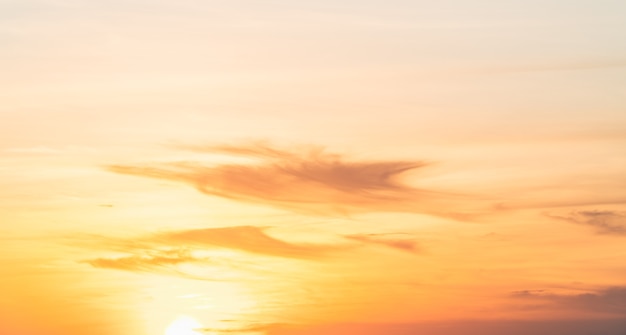The image depicts a serene and colorful sunset sky with a light grayish-blue tone at the top, gradually transitioning into hues of pink, purplish, orange, and yellow. The bottom of the sky has a dark purple tint with pink undertones. To the left, the sun's presence is indicated by a bright area with orangish clouds over it. The middle of the sky features some airy, flowing purple clouds, adding to the ethereal quality of the scene. The sun, although not fully visible, casts a brilliant whitish-yellow light source near the bottom left, where a half-circle of intense brightness suggests its setting position. This light radiates outwards, blending with the overall orange and dull pink tones of the sky, interrupted occasionally by brownish, orange-hued clouds. The photograph captures a peaceful, hazy atmosphere with wispy clouds scattered throughout, emphasizing the gentle, fading colors and the delicate interplay of light and shadow across the sky.